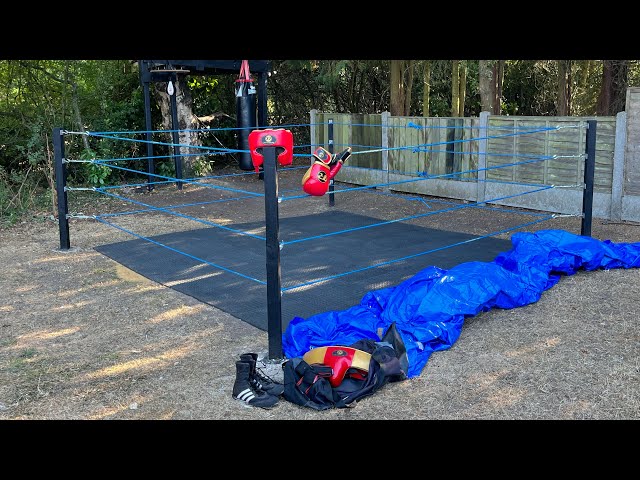This daytime photograph captures an outdoor backyard boxing ring or sparring area, distinctly framed by four metal poles with blue cord-like ropes strung between them, forming a square. The ground appears to be gravel with a mat on top. In the foreground, red boxing gloves and a helmet are seen hanging from the ropes, with two black shoes and additional scattered boxing gear strewn about. A dark blue tarp is casually pushed to the right side of the image. The backdrop includes a wooden fence running partially along the side of the ring, with trees and a forested area visible beyond the fence. No people are present, leaving the small boxing ring empty and serene.